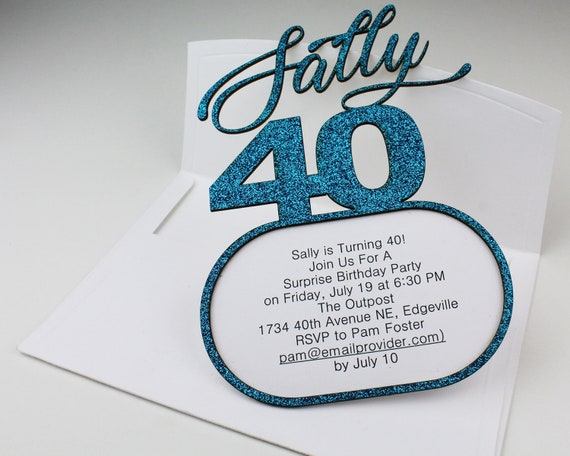Set against a clean, white background, this image depicts an elegant, glittery birthday invitation for a woman named Sally. The invitation emerges from an opened white envelope, angled to the right on a simple white surface. The invite itself is a striking blue-green hue with a glittery finish, featuring "Sally 40" in cursive at the top. Below, the text unfolds in an oval-shaped area, framed by the glittery border, and reads: "Sally is turning 40. Join us for a surprise birthday party on Friday, July 19th at 6:30 PM at The Outpost, 1734 40th Avenue NE, Edgeville. RSVP to Pam Foster at pam@emailprovider.com by July 10th." The image exudes an air of extravagance and sophistication, suitable for showcasing on a website that sells custom birthday invitations.